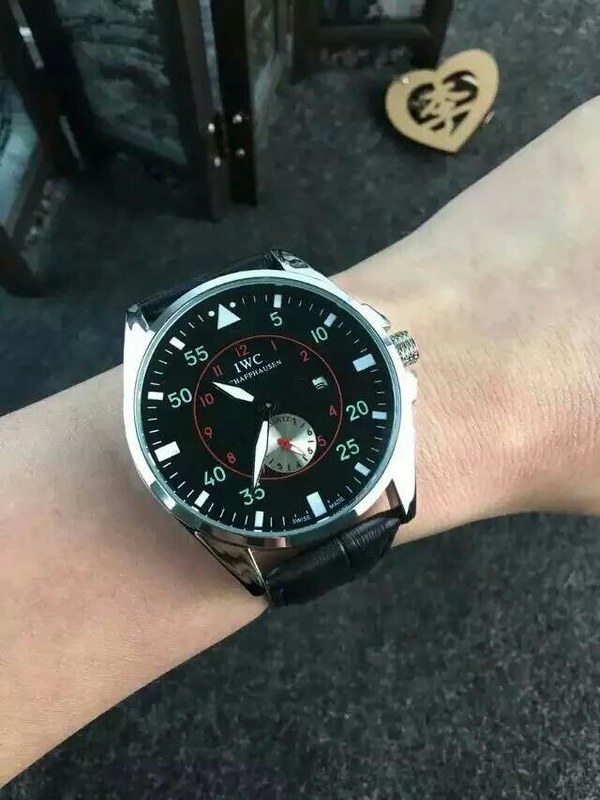The photo captures a close-up, overhead view of a Caucasian person's wrist, adorned with a wristwatch. The wristwatch has a silver-tone case and a black strap. Its black face is marked with Arabic numerals representing five-minute increments, and features rectangular markers on the outer part for these increments. The watch also includes a triangle at the 12 o'clock position and a smaller sub-dial for the seconds, positioned just below the hour and minute hands, which are white. The wrist is fair-skinned, with no visible arm hair, and is slightly tilted toward the left with the arm extending from the lower left to the upper right of the photo. In the background, there is a dark-colored or gray rug, a folding screen that appears to be an oriental privacy curtain, and a wooden or gold heart design. The watch's face indicates a time of approximately 6:52.